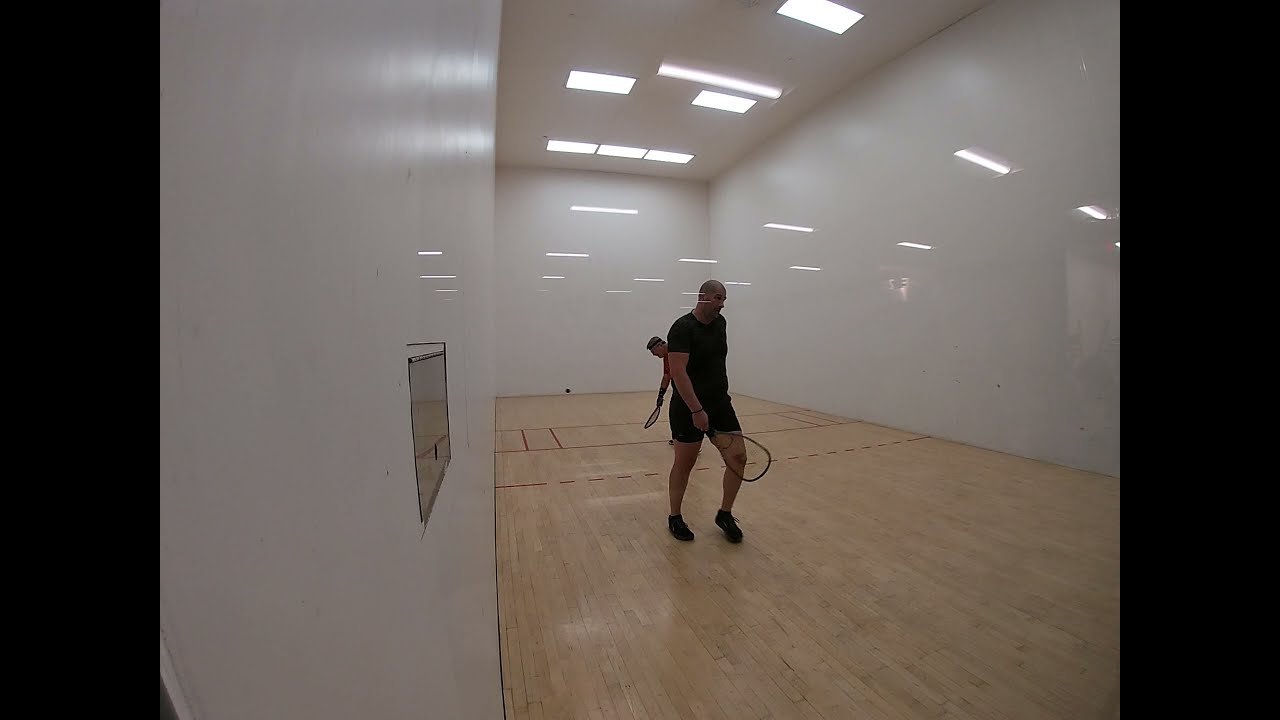This is a photograph taken indoors within a racquetball court, framed horizontally with thick vertical borders on each side, making the central image appear almost square. The room is brightly lit by numerous fluorescent lights aligned in the center of its white ceiling, whose reflections are visible on the glossy floor. The walls are uniformly white, providing a stark backdrop for the action within the court. The floor is the typical light brown with brick-shaped tiles, adorned with dashed and solid black lines marking the playing area.

At the core of the image is a bald man, or one with a closely shaved head, positioned in the middle of the court. He is dressed in a matching black outfit—black tennis shoes, black shorts, and a short-sleeved black shirt—and holds a racquet in his hand. The man appears to be walking toward the right side of the frame, possibly preparing for his next move. Directly behind him stands another player, partially obscured, bending slightly with a racquet in hand, appearing ready to serve. The setting suggests an intense one-on-one racquetball match possibly caught during a brief strategic pause. The image, captured from outside the court through the reflective glass walls, emphasizes the focused, dynamic atmosphere of this racquetball game.